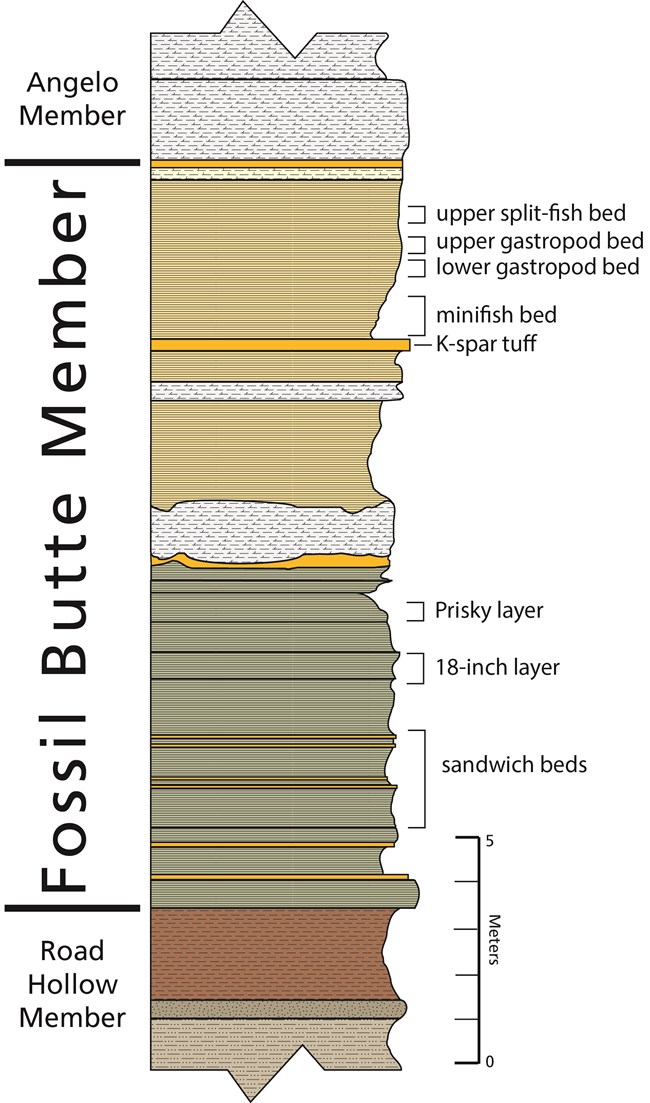The image is a detailed diagram representing different geological layers, labeled clearly on both sides and employing a variety of colors for differentiation. Along the left side, the vertical text reads "Fossil Butte Member," with "Angelo Member" at the top and "Road Hollow Member" at the bottom. The diagram’s center illustrates varying layers of earth or soil in green, brown, and tan hues, each label corresponding to a specific type or level of fossil bed. Notable layers include "Upper Splitfish Bed" at the top, followed by "Upper Gastropod Bed," "Lower Gastropod Bed," "Mini Fish Bed," "K Spar," "Tuff," "Prisky Layer," "18-inch Layer," and "Sandwich Beds." Measurements of these layers are provided in meters on the right, adding further detail to the representation of the geological strata.